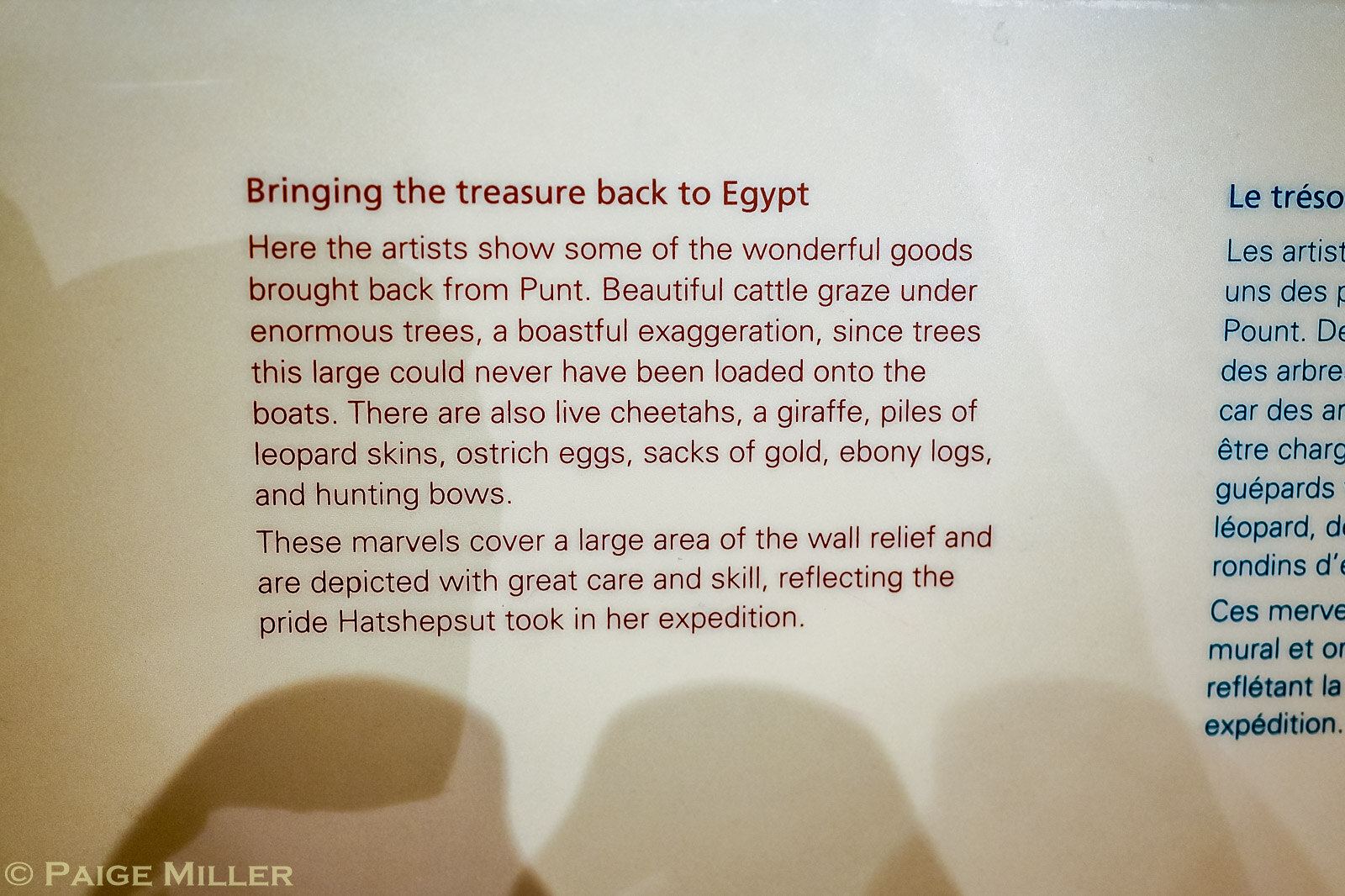This is a color photograph of an informational sign, likely from a museum display. The sign has a white background with red text prominently titled "Bringing the Treasure Back to Egypt." To the right, a translated version in blue text can be seen, although it is partially obscured. The photograph is further detailed with multiple shadows cast on the sign, suggesting several light sources behind the photographer. The text reads: "Here the artists show some of the wonderful goods brought back from Punt. Beautiful cattle grazed under enormous trees, a boastful exaggeration since trees this large could never have been loaded onto the boats. There are also live cheetahs, a giraffe, piles of leopard skins, ostrich eggs, sacks of gold, ebony logs, and hunting bows. These marvels cover a large area of the wall relief and are depicted with great care and skill, reflecting the pride Hatshepsut took in her expedition." The bottom left of the sign is marked with a copyright attribution to Paige Miller, indicated as "Paige Miller" in light text.